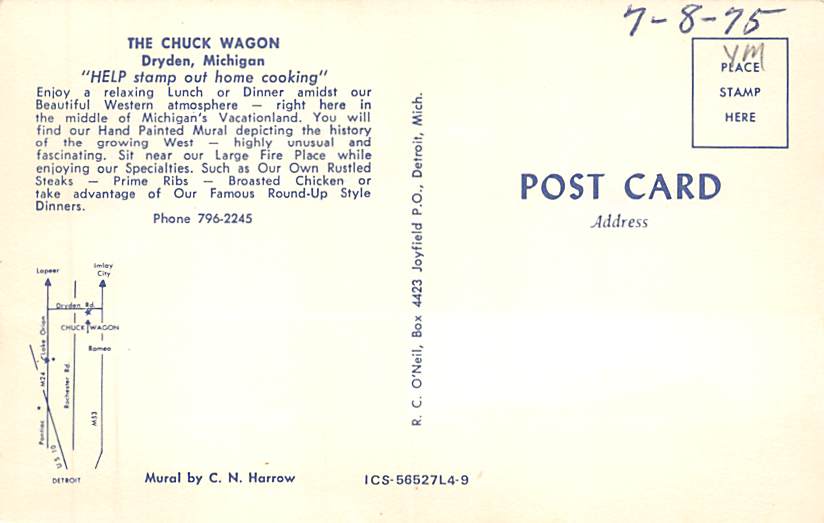This image features the back side of an aged postcard, dated 7-8-75, with handwritten initials "YM" noted above the text "place stamp here" in a blue, rectangular stamp box on the top right corner. The cream-colored postcard has browned over time, especially around the edges. On the right, in dark blue text, it says "Postcard" followed by "Address."

The left side of the postcard prominently displays text promoting The Chuck Wagon in Dryden, Michigan. The advertisement encourages visitors to "help stamp out home cooking" by enjoying lunch or dinner in a Western-themed atmosphere, right in Michigan's vacation land. Highlights include a hand-painted mural depicting the history of the growing West, alongside specialties like rustled steaks, prime ribs, roasted chicken, and famous Roundup-style dinners, all enjoyed by a large fireplace. The advertiser also provides a phone number: 796-2245.

At the bottom left, there is a simple street map marked with three vertical lines and one horizontal line, pointing to the location of The Chuck Wagon, with details written sideways in the middle, including an address. The map is accompanied by the note "Mural by C.N. Harrell" indicating the mural artist.